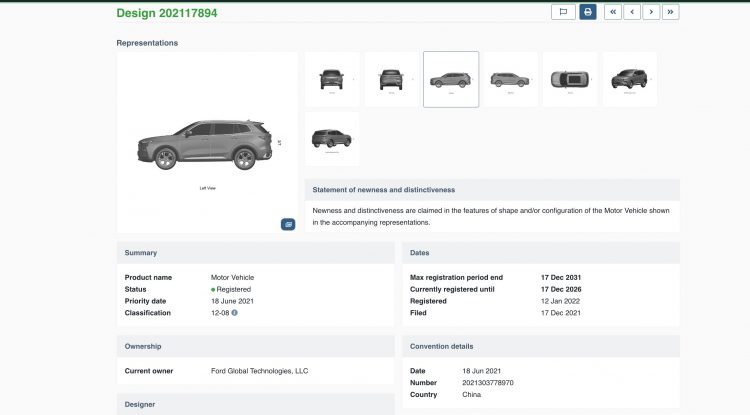In the foreground, a detailed schematic of a car is depicted, focusing on the upper left side. Prominently displayed is the text "Design 202 117 8 9 4" in green, emboldened by a green line directly above it. To the right, there is a cluster of interactive buttons, including a white button adorned with a flag, a blue button whose function remains unclear, and additional buttons marked with left and right fast-forward arrows. Below this button cluster, the word "Presentations" is poised above a gallery of eight photos of the car. Among these, seven are small thumbnails, while one image stands out larger and is framed by a square, indicating it is selected or highlighted.

Further details are arrayed in a structured format beneath, commencing with the section titled "Summary." The summary specifies:
- Product Name: Motor Vehicle
- Status: Registered
- Priority Dates: 18 June 2021
- Classification: 12-08
- Ownership: Current owner is Ford Global Technologies LLC
- Designer: Not specified

On the right side, additional important dates and registration details are listed:
- Mass Registration Period Ends: 17 December 2031
- Current Registration Entailed: 17 December 2026
- Registered: 12 January 2022
- Filed: 17 December 2021
- Convention Details: Date 18 January 2021